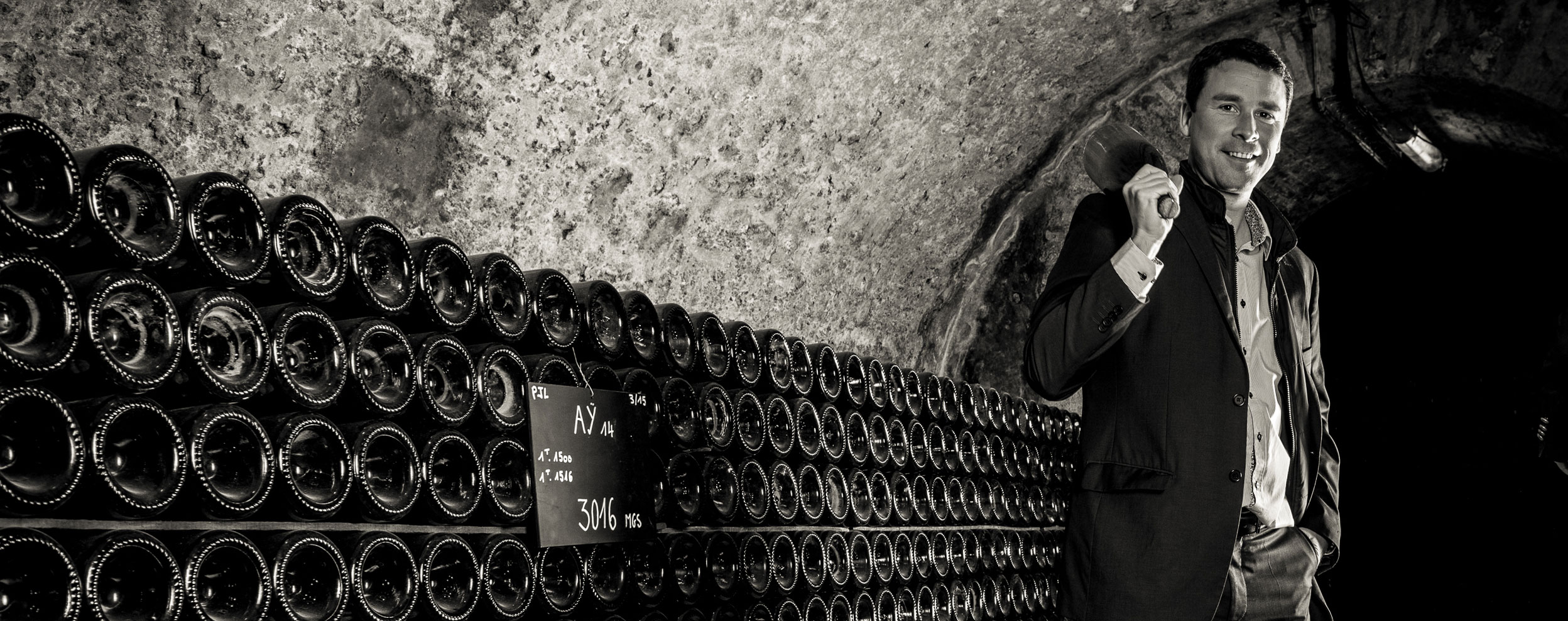This black and white photograph features a man standing in a wine cellar. He is wearing a black dress coat, dress shirt, and dress pants, and he has short, dark hair. The man is smiling at the camera while holding a bottle of champagne over his right shoulder in his right hand. Behind him, there is an extensive wall lined with numerous wine bottles. The background includes a rounded light gray wall above and a dark section on the right. Text and numbers are visible on the wine bottles, including "2016." The setting suggests an aged, atmospheric wine cellar with an electric light hanging from the ceiling, casting shadows on the weathered walls marked with holes and signs of aging. The photo appears professionally staged, capturing the celebratory and timeless ambiance of the cellar.